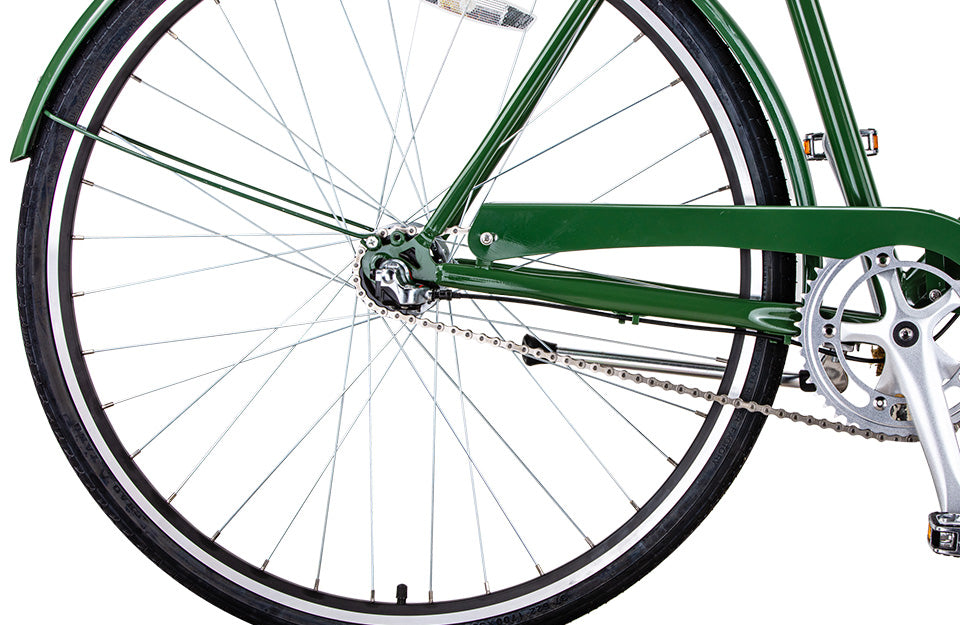This close-up photograph showcases the back wheel of a meticulously polished, green-framed bicycle. The frame's metallic finish shines brilliantly under professional, soft, and even lighting. Set against a pristine white background, the image highlights the bike's minimalistic yet elegantly designed transmission system, reminiscent of a classic style. The wheel, occupying approximately 90% of the frame, partially extends beyond the image's boundaries. A safety-reflective strip is also visible on the wheel, underscoring the bike's thoughtful design for both aesthetics and safety.